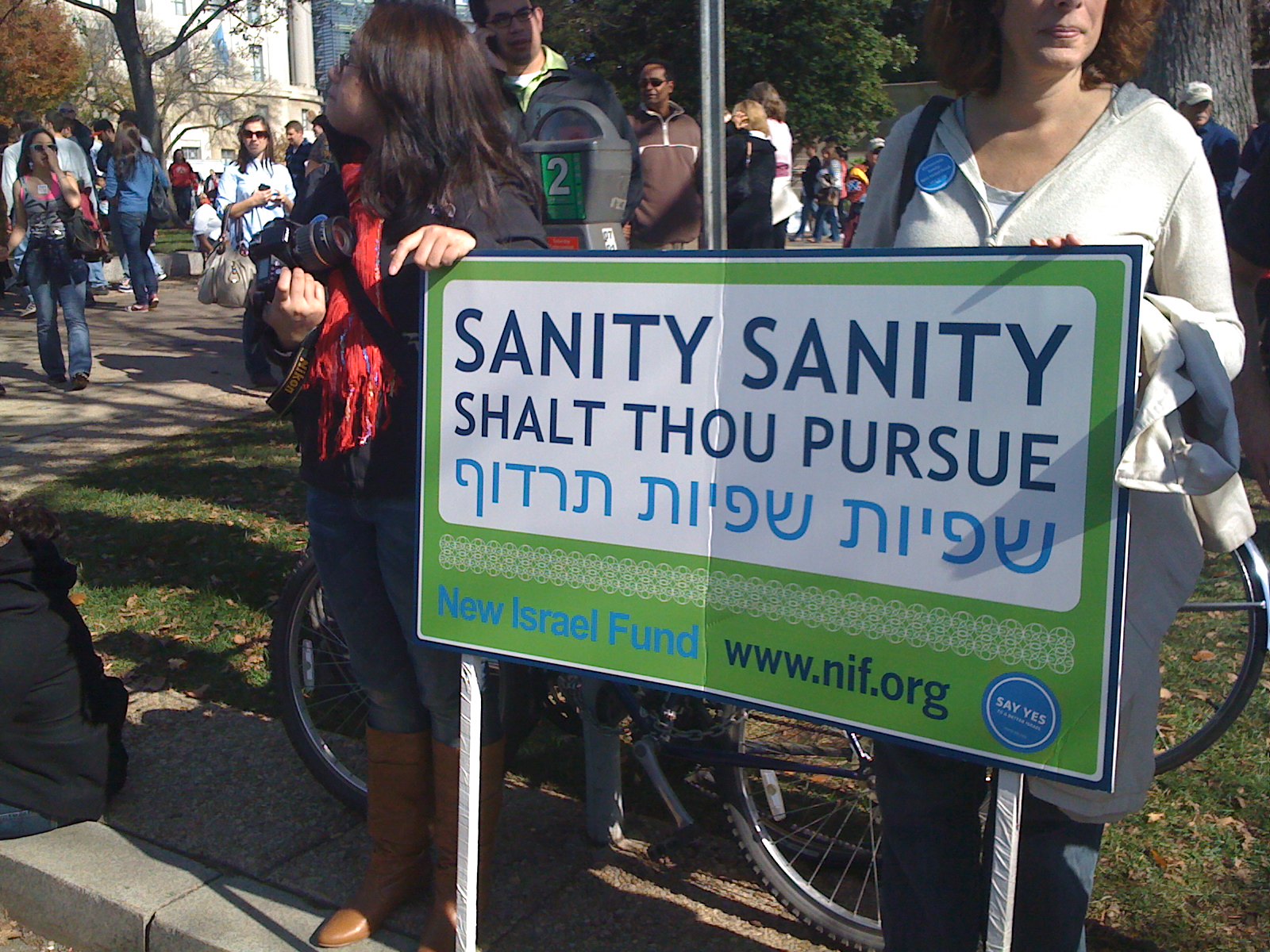The image depicts an outdoor scene with two women holding a large rectangular sign mounted on two poles. The sign, which has blue and green borders, reads "Sanity, Sanity, thou shalt pursue" in blue text on a white background, with Hebrew writing underneath, likely "Shafit Tradif." Below the text, it says "New Israel Fund" along with the URL "www.nif.org," and features a blue circle with "Say Yes" inside. The women are positioned on a concrete sidewalk in what appears to be a town or city area with a park-like setting. The woman on the left is wearing a black sweatshirt, blue jeans, and light brown leather boots, and she holds a camera with a large lens. The woman on the right, possibly older, is dressed in a white sweatshirt and navy pants, and they seem to be participating in some form of gathering or protest. The background includes multiple people, bicycles, and a mix of stone and dark buildings with many windows, giving the area a college campus or town square feel. There are trees with brown leaves and a grassy yard, contributing to the overall autumn atmosphere.